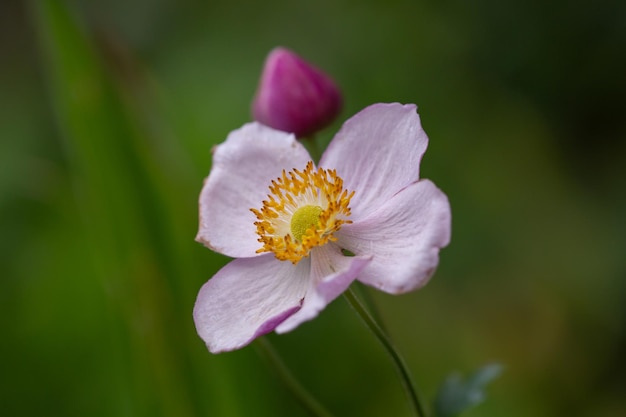This image is a professionally taken, aesthetically pleasing close-up photograph of a delicate flower with intricate details. The flower, with its five lilac-colored petals that have a faint hint of purple or pink, is the focal point and is captured in sharp focus, revealing the fine wrinkles and textures of each petal. At the core, there is a lime green center encircled by tiny, vibrant yellow stamens. Near the flower’s base, a green stem with visible fuzz supports the bloom. Just behind the main flower is an unopened bud, resembling a small, dark purple plum or an inverted tulip, hinting at a potential flower yet to blossom. The background contrasts beautifully, rendered in various blurry shades of green, possibly indicating surrounding leaves or grass, providing a natural, serene setting without any text present.